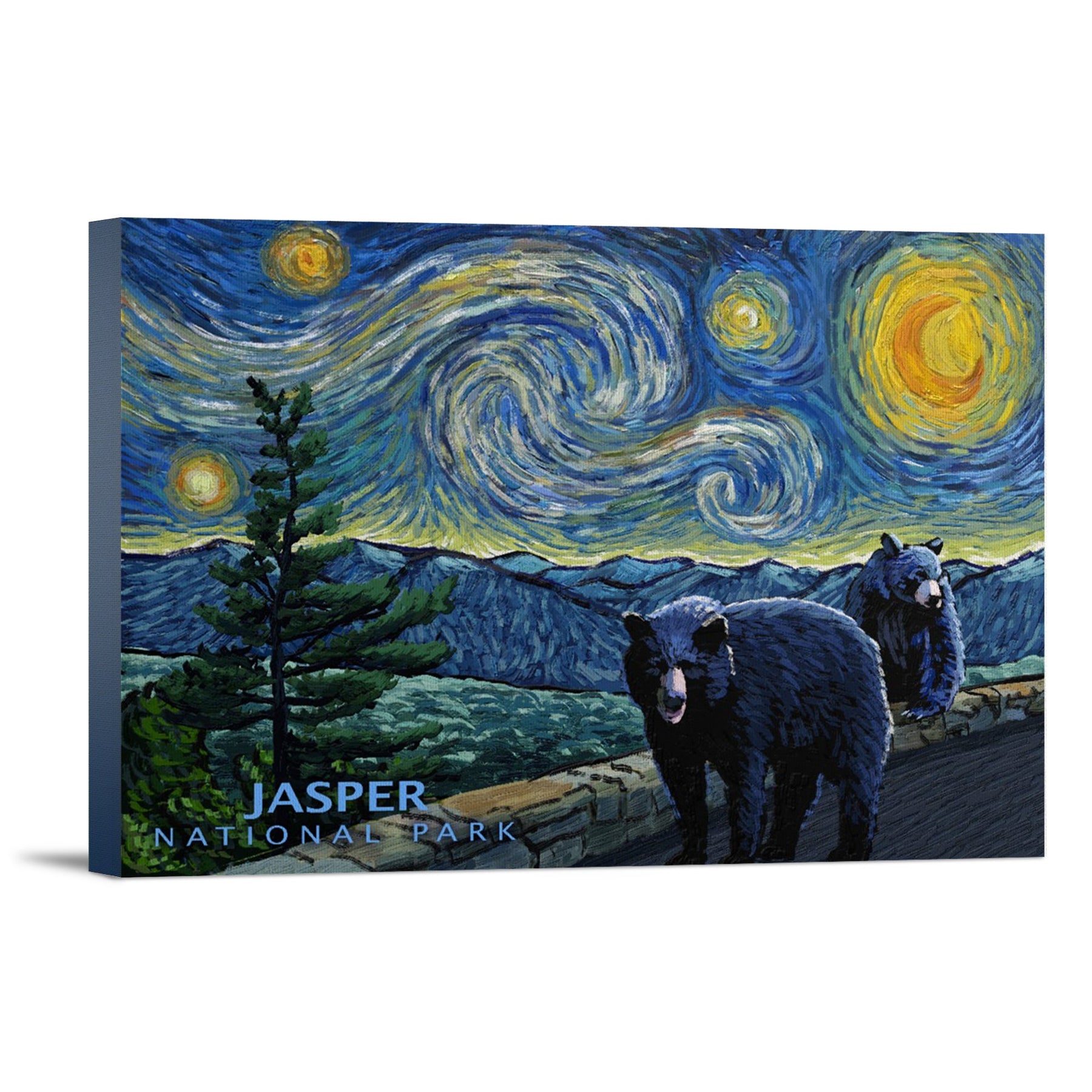This image appears to be an artistic homage to Van Gogh’s famous painting "Starry Night," yet it incorporates unique elements that set it apart. The sky features the iconic swirly blue and yellow patterns reminiscent of Van Gogh's masterpiece, creating a striking and beautiful visual effect. However, instead of a village scene, the foreground showcases majestic mountains and a winding road. Notably, there are two black bears; one bear is on all fours while the other sits upright on a ledge by the road, and both are intriguingly looking directly at the viewer. The scene is framed by several pine-like trees, adding to the natural ambiance. In the bottom left-hand corner of the painting, the words "Jasper National Park" are inscribed in blue, suggesting the artwork serves as an advertisement for the park. The overall color scheme prominently features yellows and blues, accentuated by the green of the trees, contributing to the painting’s vivid and vibrant appeal.